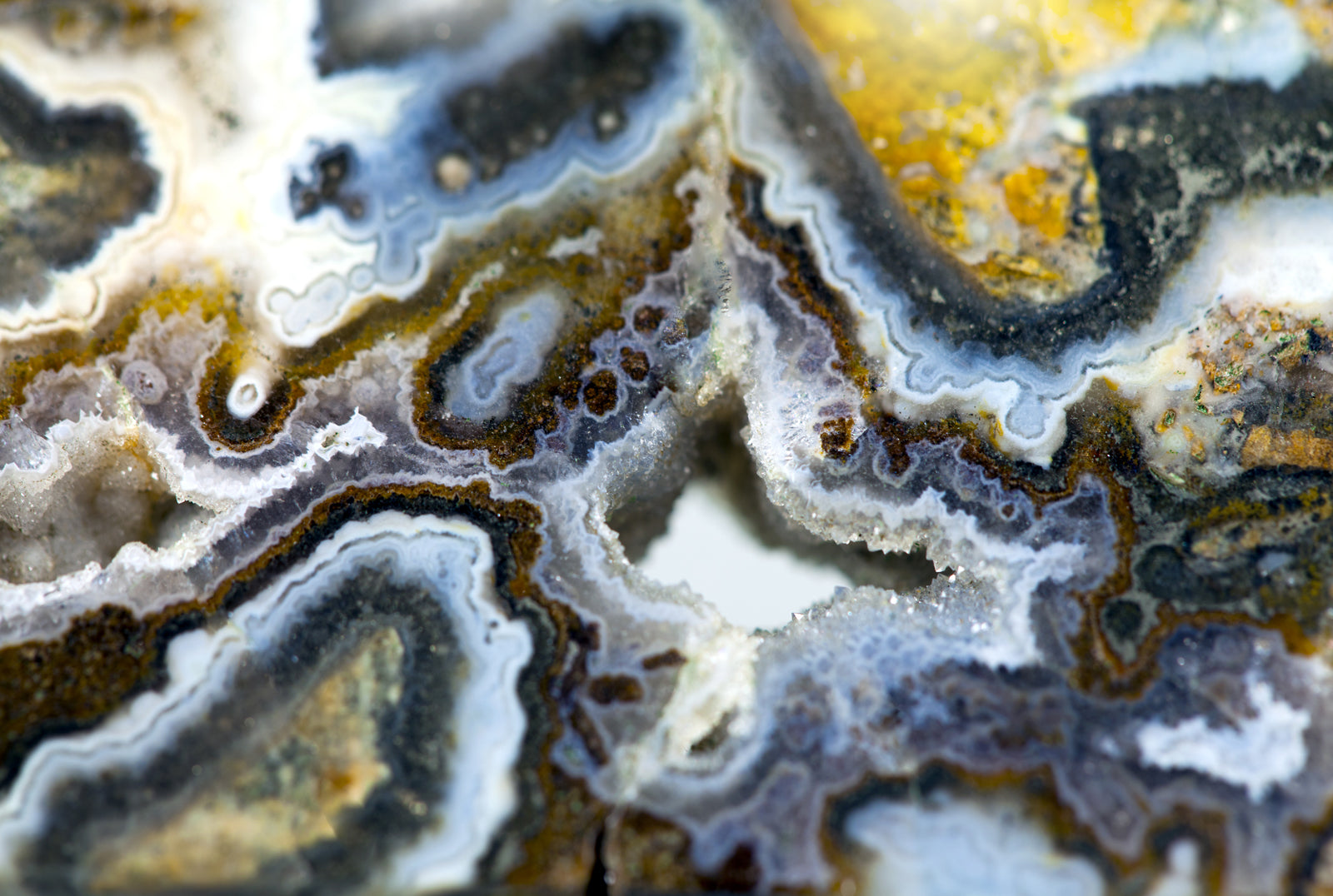This is a highly detailed, close-up photograph of a cross-section of a geode-like rock, which has been cut into a flat plate and polished. The photo reveals an intricate tapestry of colors and layers. The outermost layer is a dark brown, followed by successive irregular layers of white and light blue. Further in, there's a light blue layer, surrounding a core of multi-colored substance comprising yellow, blue, and brown particles. The top-right section of the image features a prominent bright yellow patch. Swirling patterns dominate the structure, and several irregularly shaped holes run through the rock, lined with sparkly, clear crystals. The overall composition of the rock is chaotic yet mesmerizing, displaying a remarkable blend of colors including yellows, olive greens, light blues, blacks, whites, and various shades of brown.